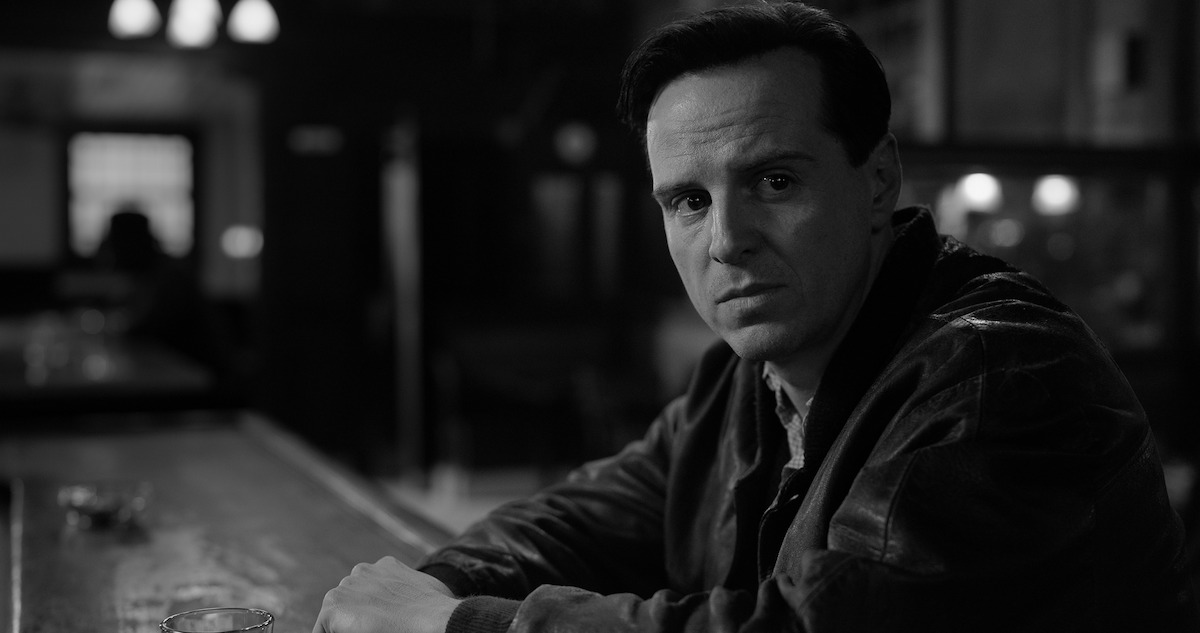In this black and white screenshot from the Netflix series "Ripley," actor Andrew Scott is seated at a wooden bar counter, embodying a vintage, old-movie aesthetic. Dressed in a black leather jacket, he gazes to the right with a concerned expression on his face, his dark hair and intense focus adding to the scene's dramatic tension. His hands rest thoughtfully on the bar's surface, where a small shot glass sits slightly off to the left. The background, a dimly lit interior with a dark green hue, is beautifully blurred, drawing attention to Scott's character who is illuminated by brightly lit lights that cast a crisp white glow over the entire scene.